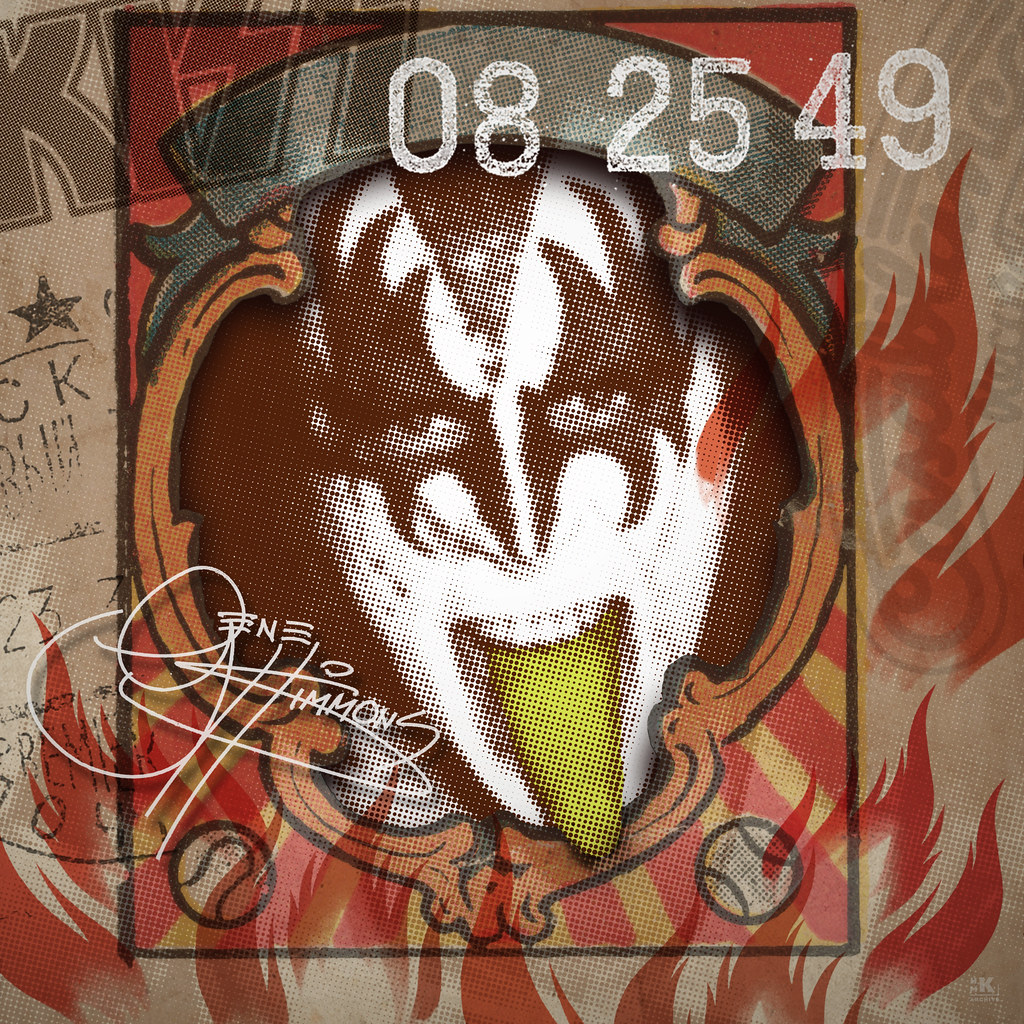This image captures a striking portrayal of Gene Simmons from the band KISS, set against a beige background. Featured prominently is a large, black-trimmed square with bold orange edges, adorned by vivid red flames licking upward from the bottom and right sides. Inside the square, the centerpiece is Gene Simmons’s face, iconic for its dramatic makeup: a white face paint with an intricate black design forming a mask-like pattern around his eyes and extending into points. A distinctive, oversized green tongue juts out from his mouth, contrasting with his bright white teeth. Notably, a hint of red graces his left cheek. At the top left of the image is the KISS logo, while the numbers "082549" are stamped conspicuously at the top. Additional details include a signed imprint of Gene Simmons's signature in white text. Scattered within the composition are sporting icons, including what looks like a baseball, enhancing the eclectic and vibrant nature of this poster-like display.